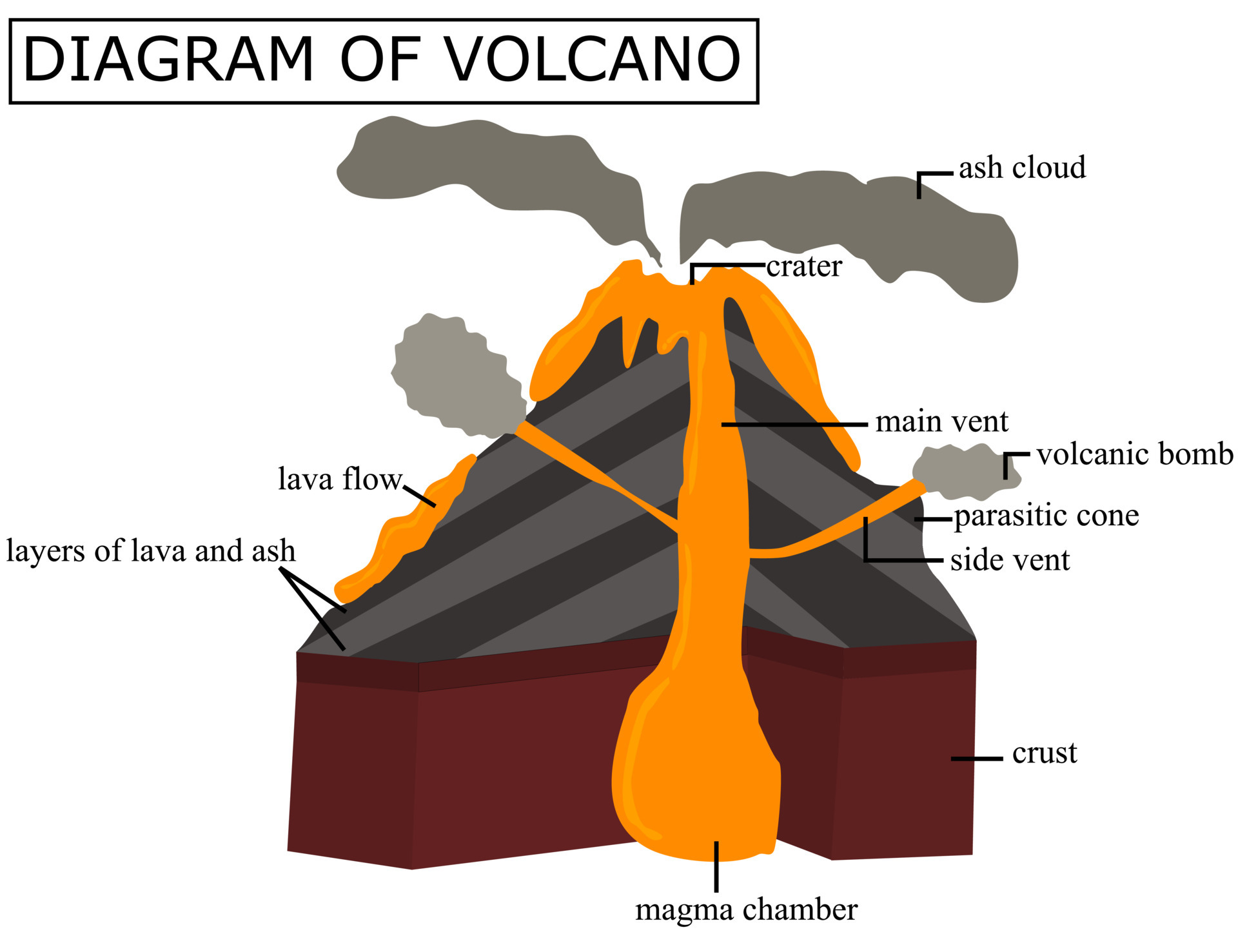The image is a detailed diagram of a volcano set against a white background. In the top left corner, enclosed in a black-outlined rectangular box, it reads "Diagram of a Volcano" in bold lettering. The central illustration is of a volcano, with its base depicted in dark brown representing the crust. An inner section at the bottom center labeled "Magma Chamber" indicates where magma is stored beneath the surface.

The volcano's structure includes gray and dark gray layers signifying "Layers of Lava and Ash." These layers are angled upwards, converging at the volcano's peak. Bright orange lava is shown flowing from the crater at the top and labeled "Lava Flow," cascading down to the bottom of the image. At the apex, two gray ash clouds emerge, with labels "Ash Cloud" in black text positioned near each cloud, indicating their dispersion to the left and right.

The diagram also includes multiple labeled components: "Main Vent" points to the vertical channel through which magma travels, while "Crater" denotes the opening at the summit. "Side Vent" and "Parasitic Cone" labels highlight additional pathways and smaller cone structures on the sides. Additionally, there is a label "Volcanic Bomb" marking the ejected solid fragments during an eruption.

Overall, this thorough diagram depicts the intricate structure and various elements of a volcano, clearly marked and labeled for educational purposes.